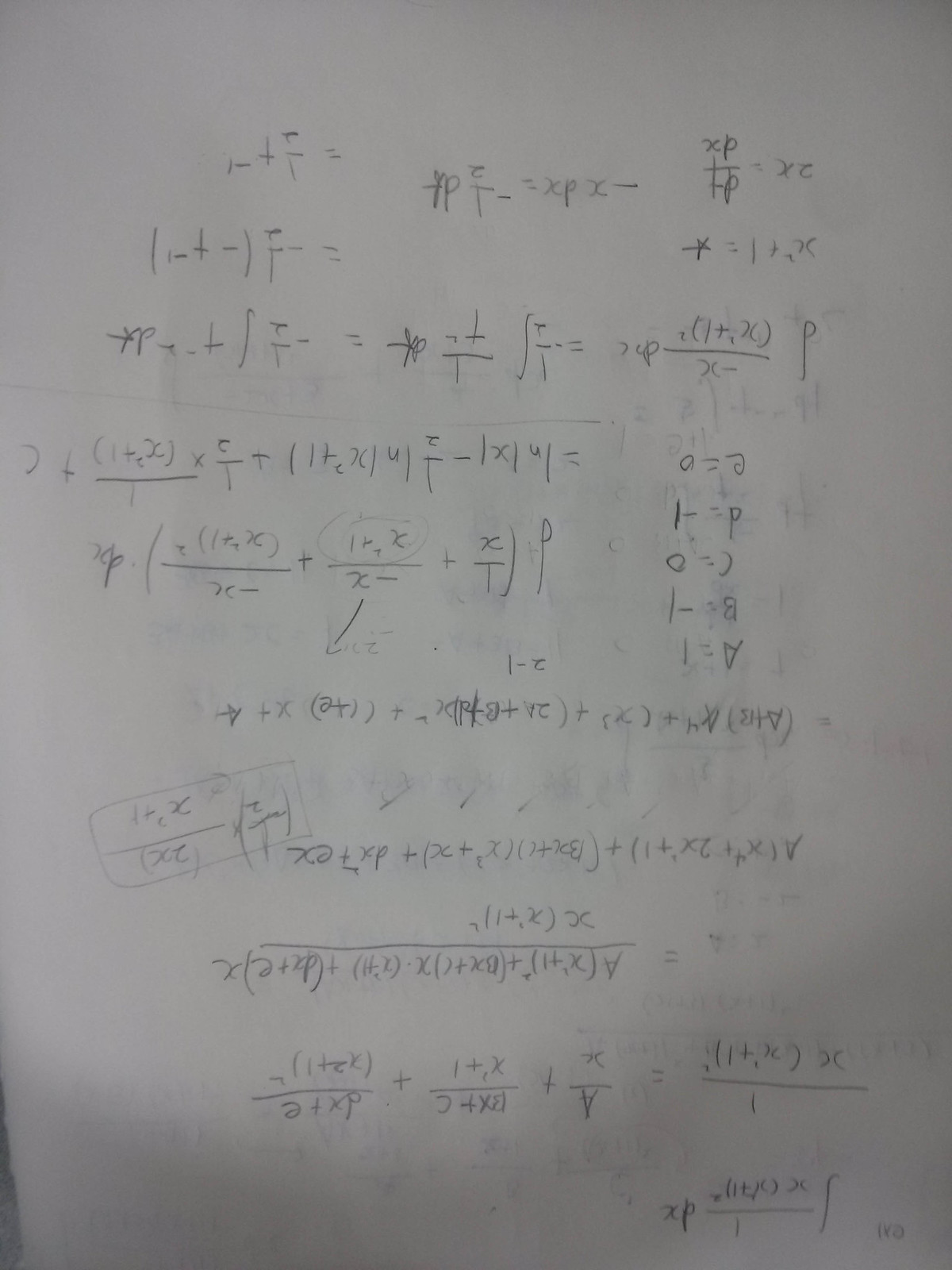This image depicts a standard white sheet of paper laden with intricate mathematical equations. The equations are arranged in multiple horizontal rows, indicating methodical problem-solving. The paper appears to be oriented upside down, providing a unique perspective on the mathematical work. The notations include an abundance of variables, predominantly 'X' and 'C', suggesting algebraic and possibly calculus-based complexities. Among the equations, there are instances of fractions, such as expressions involving '1/X'. 

Roughly halfway down the page, oriented to the right due to the inverted view, a series of variables are defined: A=1, B=-1, C=0, D=-1, and E=0. These values likely play pivotal roles in solving the overarching mathematical problems presented on the sheet. Despite the challenging orientation, the meticulous and structured nature of the work is apparent, showcasing a deep engagement with advanced mathematical concepts.